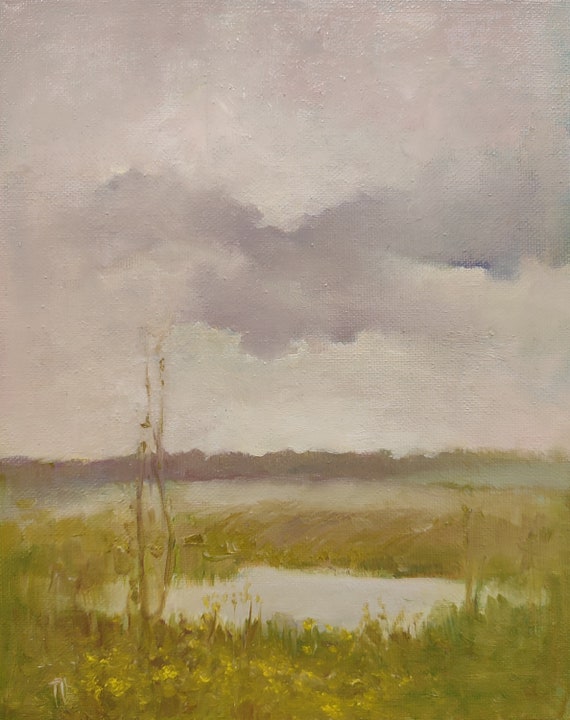This painting, with its textured and runny details suggesting a watercolor or oil-based medium, depicts a moody, overcast day in a wetlands or swampy area. The sky, occupying two-thirds of the canvas, is dominated by stormy clouds ranging from light to dark gray. In the distance, a shadowed outline hints at a tree line. The foreground features an overgrown field of shaggy, bushy grass in shades of green and brown, interspersed with small, faint yellow wildflowers. At the center bottom, a small, oval-shaped pond reflects the gray sky above. To the left corner, a tiny sapling stands bare, adding to the scene's somber, reflective mood.